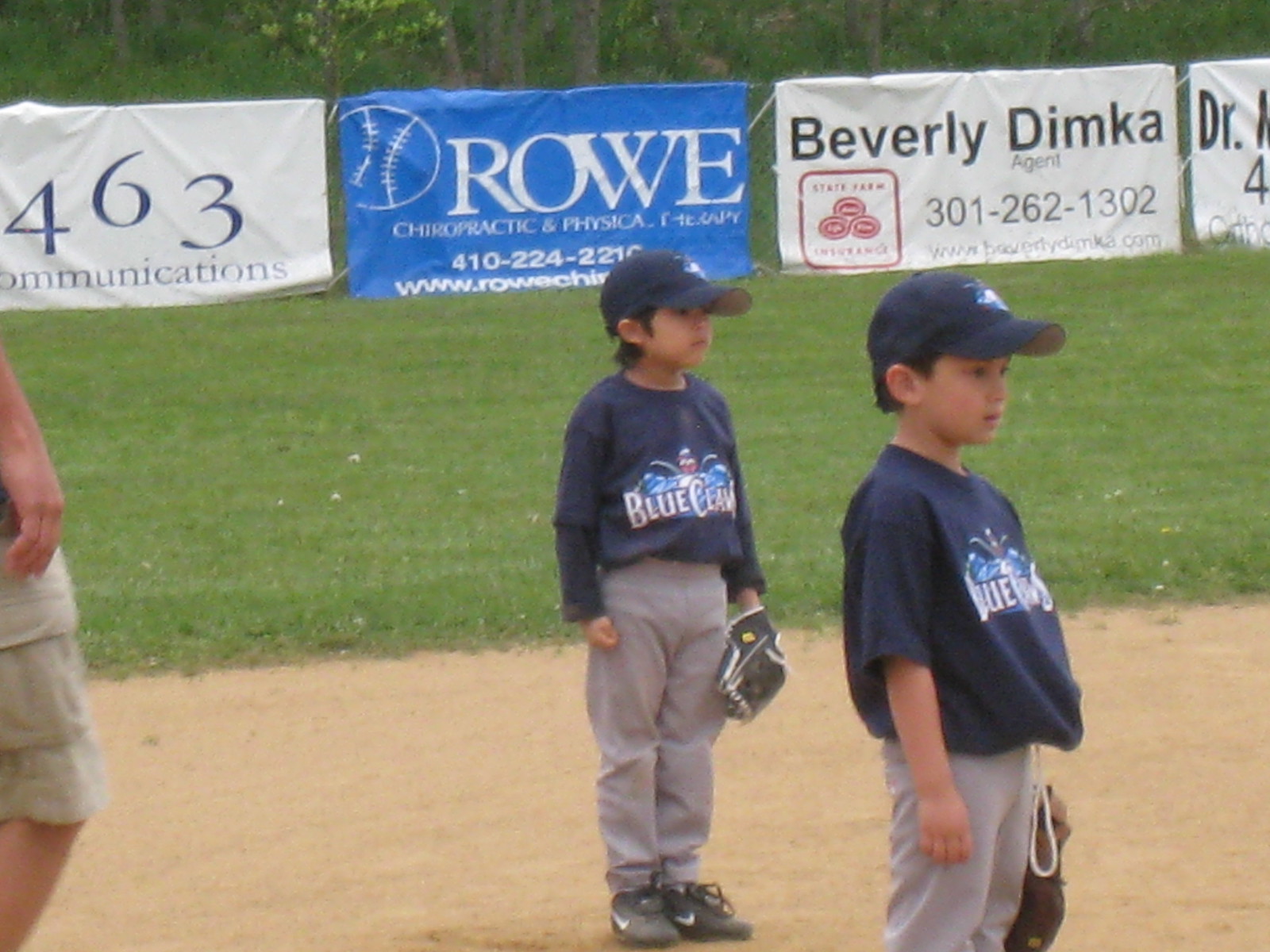In the image, two little boys stand straight and attentive on a brown baseball diamond, poised as if about to start a ball game. Dressed in navy blue sweatshirts emblazoned with "BLUE MAYBE CREEK" and matching baseball caps, they each hold a baseball mitt. The boys, positioned in the center of the frame, are clearly the main focus of the picture. The setting appears to be a Little League baseball field, with green grass and a chain-link fence visible in the background. Attached to the fence are several advertisement signs, including one for "ROW PHYSICAL THERAPY" with a phone number, a large blue sign, and another for "BEVERLY DIMKA" alongside an All-State logo and contact details. To the right, a partially visible sign mentions a "DOCTOR." On the left edge of the frame, almost out of range, is an adult’s leg, suggesting the presence of a supervising figure. The colors in the image span from tan and brown on the ground to various shades of blue, green, and white, indicating a bright, daylight setting. The background features greenery with trees and shrubbery casting a dark green shade, enhancing the outdoor ambiance.